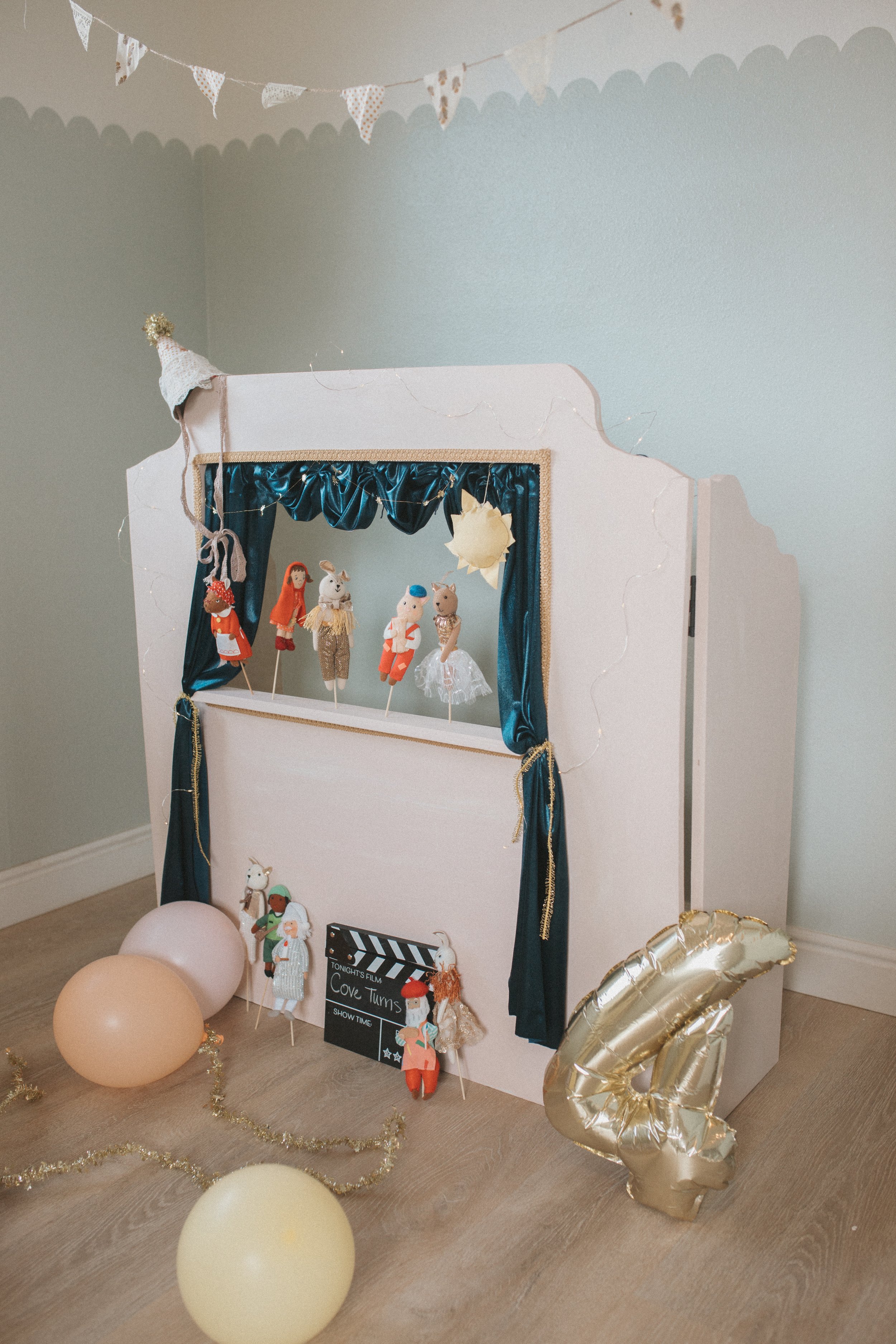The image is a full-color, meticulously staged indoor photograph featuring a puppet theater setup. The background showcases light teal-blue walls with white molding at the floor's edge, and the ceiling appears white. There is a wooden baseboard along the floor, which is composed of light-colored wood planks. Across the top of the scene, a festive banner with white polka-dotted triangular flags hangs.

Central to the image is a wooden puppet theater designed with a trifold panel, creating a semi-enclosed backstage area. The main panel features a rectangular stage window framed by dark blue silk curtains that extend nearly to the floor. A variety of colorful puppets on sticks are visible on the stage, including characters resembling Little Red Riding Hood, a rabbit, a pig, and a reindeer in a dress. Hanging from the curtains is a sun prop, adding to the whimsical atmosphere.

The floor is scattered with several balloons, including a prominent gold one that displays the number "four," suggesting a birthday celebration. Additional props include a Hollywood-style clapperboard positioned near the theater, enhancing the playful and theatrical theme of the setup.